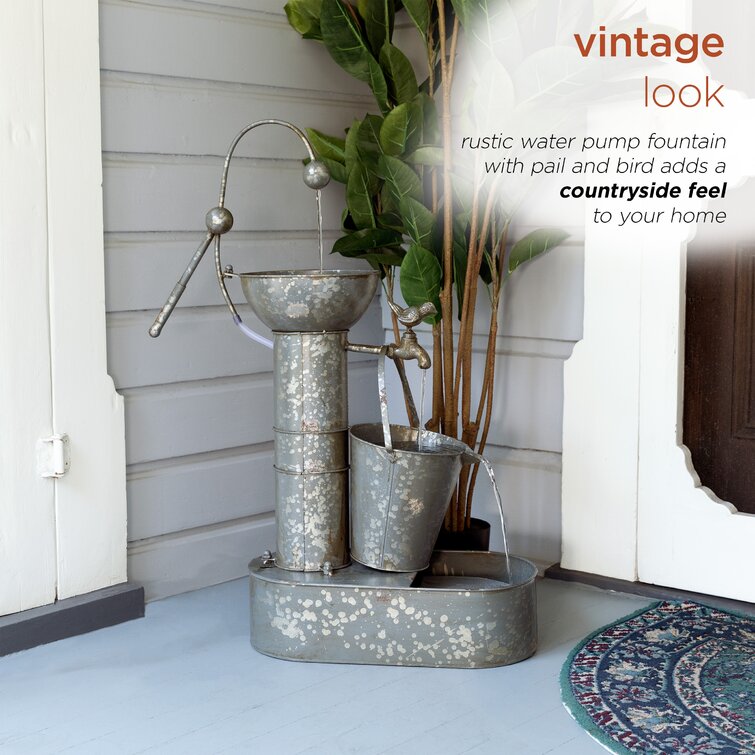The image appears to be the cover of a magazine, showcasing a decorative, rustic water pump fountain with a pail and a bird, designed to add a countryside feel to your home. This actual pump fountain is front and center in the photograph. It is constructed from metal and sits on a gray hardwood floor with a gray background, complemented by a wooden backdrop. Studio-grade lighting enhances the image's starkness, highlighting the pastel colors like gray, light blue, and green throughout.

In the top right-hand corner, inset text reads "Vintage Look" in orange, followed by "Rustic water pump fountain with pail and bird adds a countryside feel to your home" in black lettering. A small throw rug or welcome mat lies at the bottom right portion of the image.

Situated on what appears to be a front porch, the scene includes a door to the right with glass panes and blue carpeting, while to the left of the fountain, a partially visible white door with a hinge suggests functionality. A potted plant is placed behind the fountain, and the overall setting is designed to evoke a charming, rustic aesthetic.